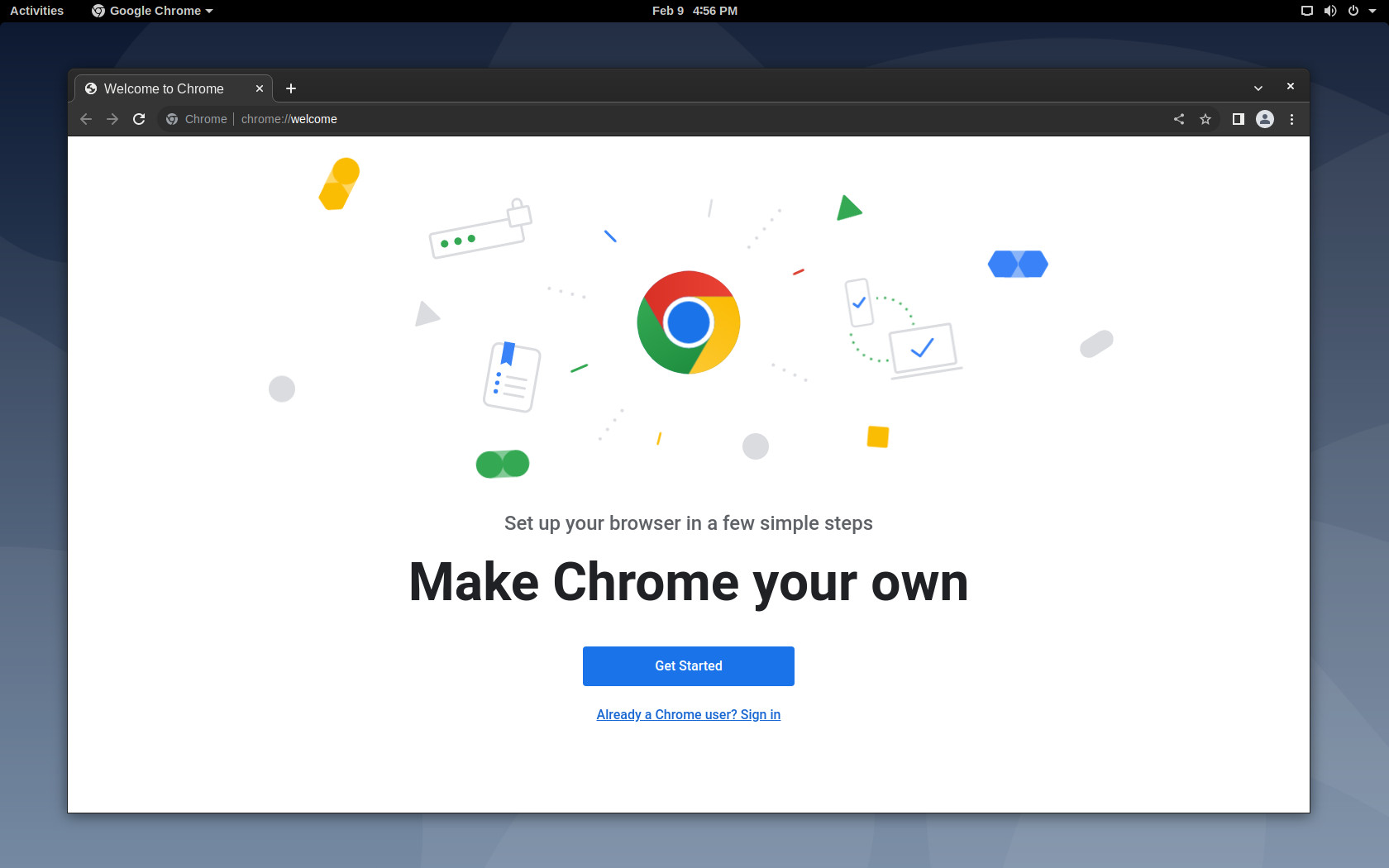The image features a web page displayed in a browser, with a focus on setting up Google Chrome. The central part of the screen showcases text that reads, "Set up your browser in a few simple steps. Make Chrome your own." Directly below this message is a prominent blue button with white text that says, "Get started." Underneath this button, there is a blue hyperlink stating, "Already a Chrome user? Sign in."

Above this central text, an iconic Google Chrome logo is displayed. The logo consists of a circular design with three outer segments in red, green, and yellow, and a central blue circle. A white outline separates the outer and inner sections of the logo.

Surrounding the main content are various graphical elements, including green triangles, yellow squares, gray circles, gray triangles, and icons of devices with checkmarks, suggesting synchronization. On the top left corner, there is an icon of a password lock in green and gray colors. At the bottom left, a series of green circles are connected together.

The background of the entire image is white. At the top left, the text reads, "Welcome to Chrome," corresponding to the URL shown as "chrome://welcome," which is displayed in black against a white background.